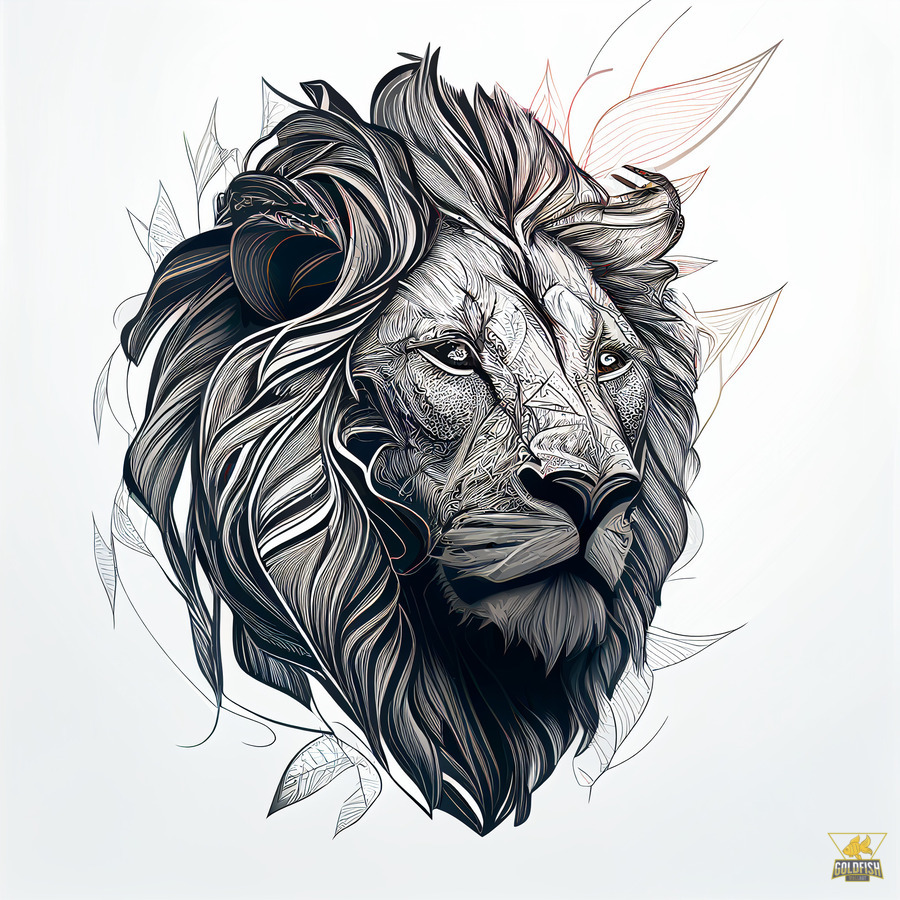This intricately detailed black-and-white drawing showcases the majestic face of a lion, staring off to the right, with its full and elaborate mane encircling the face. The artist has used a multitude of fine lines to meticulously craft the lion's fur, especially prominent on the forehead to the nose. Leaves are interwoven with the mane, giving an impression of the lion being partially composed of plant elements. The lion’s eyes are pale and empty, adding a haunting allure, and the nose starkly black, acting as a focal point amidst the detailed facets of its face. Behind the lion, faint and indistinct lines serve as a backdrop, while a subtle hint of reddish-purplish tint appears in the upper right portion, adding a touch of color to the otherwise monochromatic scene. The background is a very light gray, providing a contrast that highlights the complexity of the lion’s features. In the bottom right corner, there is a watermark featuring a small triangle with a goldfish inside it, accompanied by the word “goldfish” beneath the drawing.